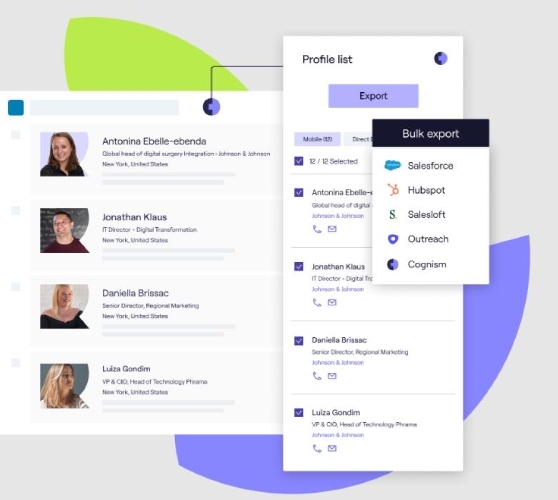The image depicts a multi-layered presentation slide from a business application. In the background, there's a brand symbol that features a green leaf and a blue wedge. Overlaid on this background, the second layer displays a list of employees, including Antonina, Jonathan, Daniela, and Louisa, along with their respective job titles such as IT Director and Senior Director of Regional Marketing. The third layer highlights a profile list showcasing various contacts with an "Export" button prominently featured. The topmost layer captures the action of someone clicking the "Export" button, revealing options for bulk exporting contacts to platforms like Salesforce, HubSpot, SalesLoft, Outreach, and Cognizant. This illustration suggests the ease of managing and exporting business contacts through the application.